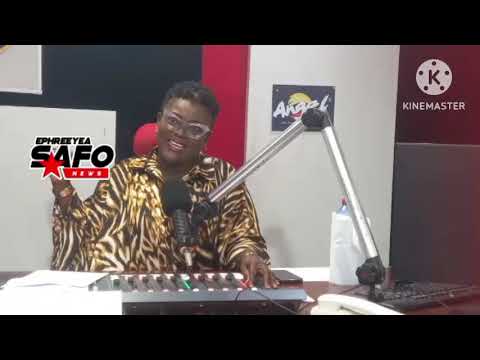The image captures an African American woman seated at a desk in what appears to be a studio or sound booth. Behind her, the wall is decorated with geometric shapes in a palette of grays, blacks, reds, and whites, featuring a picture labeled "Angel" and a gray circle with a maroon "K" and three dots, accompanied by the text "KINE MASTER." She is wearing large, semi-transparent butterfly-rimmed glasses, which appear pink or silver, and has very short curly black hair. Her attire is a loose-fitted, tiger-striped blouse with a collar and buttons. The woman is engrossed in her work, manipulating a knob on an audio switchboard with her left hand while her right hand is raised, caught in mid-gesticulation. Positioned under her mouth is a large microphone attached to an articulating stand that extends upwards and then downwards from its joint. Her mouth is open, suggesting she is speaking or singing. To the left of her, there is text reading "E-P-H-R-E-E-Y-E-A, S-A-F-O" with a red star over "S-A," followed by "News." Additionally, a black header and footer outline the image, indicating it may be a screenshot from a TV show or social media.